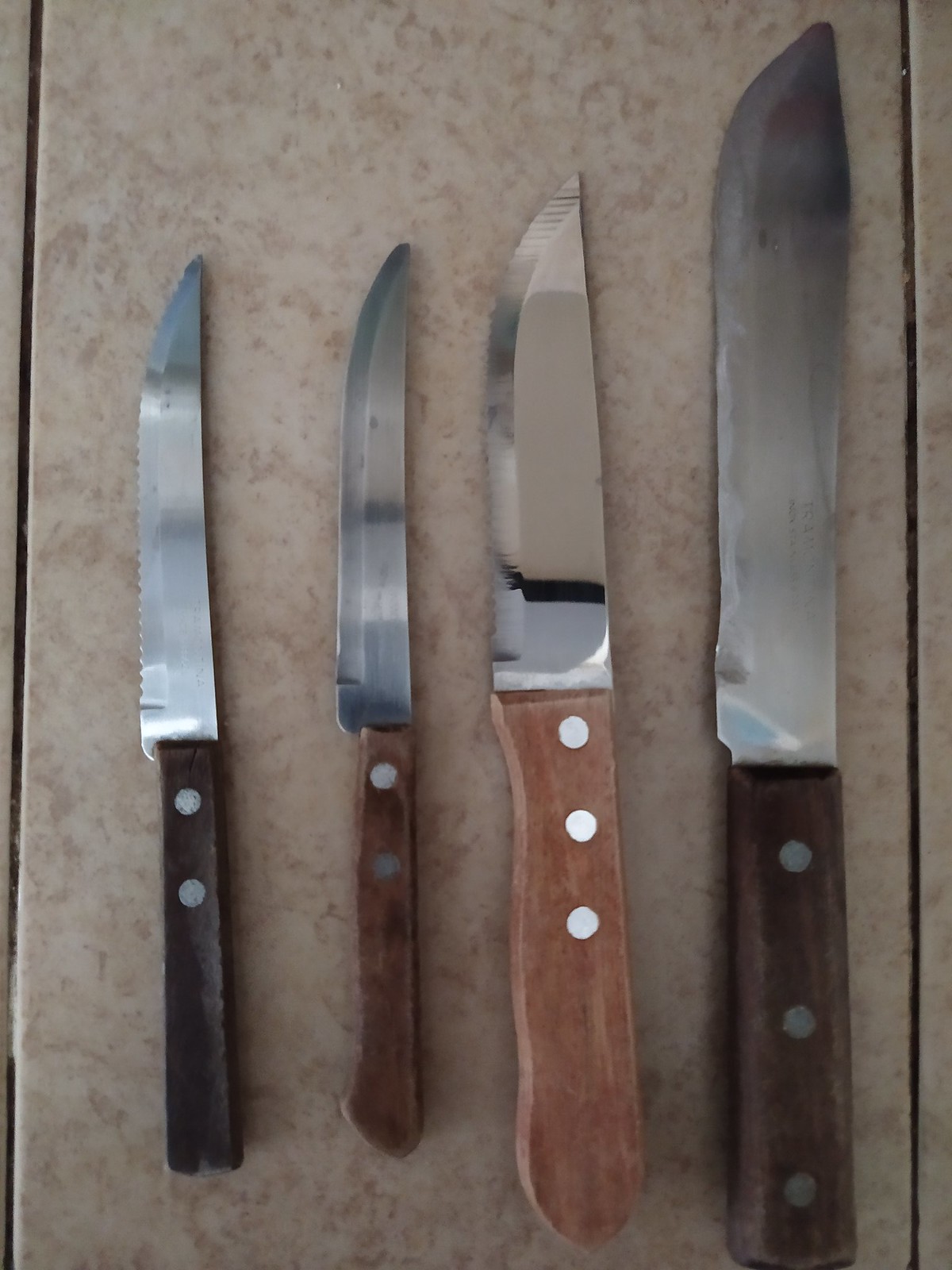This photograph features four knives meticulously arranged side by side on a beige, mottled marble or ceramic tile backdrop. The image is in portrait orientation, with the knife handles positioned at the bottom and the blades pointing upward. 

From left to right, the knives are as follows:

1. The first knife is a smaller, thin steak knife with a dark brown handle featuring two silver rivets. Its blade is slightly serrated.
2. The second knife, similar in size to the first, has a medium brown wooden handle with two silver rivets. Its blade is smooth and non-serrated.
3. The third knife is larger and has a lighter brown wooden handle with three silver rivets. This blade is slightly wider, shinier, and appears to have a mild serration.
4. The fourth and final knife is a cleaver, distinguished by its tall, wide blade that appears dinged and well-used. It has a dark brown handle with three silver rivets.

Each knife's curved edge is oriented to the left, creating a visually intriguing layout that highlights the subtle differences in design and wear.